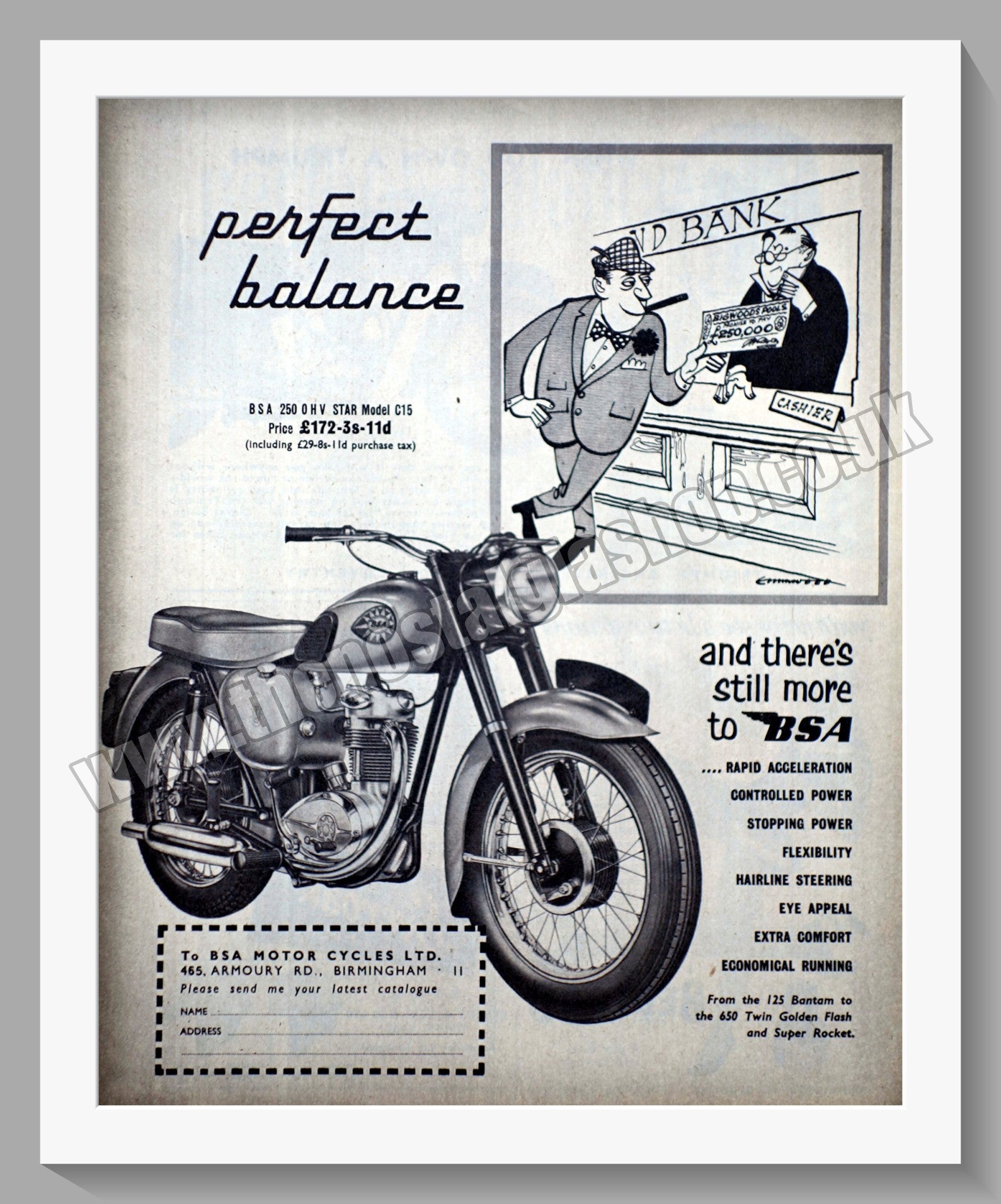This advertisement, likely from the 1950s, showcases a brand-new PSA motorcycle in a black and white image. Prominently featured on the left side, the motorcycle is highlighted against a backdrop of technical specifications detailing its rapid acceleration, controlled power, stopping power, flexibility, hairline steering, eye appeal, extra comfort, and economical running. The upper left corner features the phrase “perfect balance” in cursive script. In the upper right corner, there's a cartoon image of a man handing a large check to a bank cashier behind a window labeled "bank," possibly illustrating the purchase process. The ad's lower right corner includes additional text emphasizing the bike’s exceptional features and the phrase “and there's still more to BSA.” A watermark across the image reads, www.postalshop.com.uk, indicating availability from this online store. The advertisement also includes a coupon section at the bottom for potential buyers to clip out, fill in their information, and mail in.